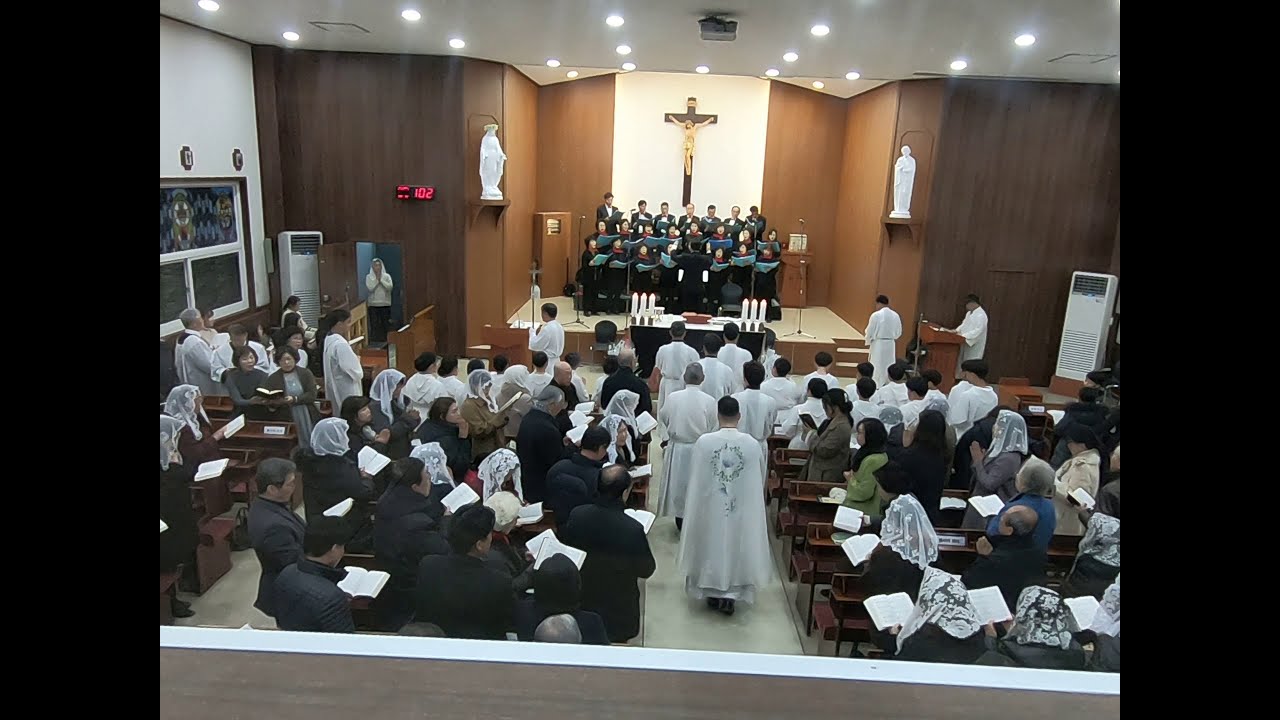This photograph captures a vibrant church service, taken from an elevated viewpoint at the back of the church, looking down the middle aisle toward the altar. The scene is set within a Catholic church, evidenced by the large crucifix with Christ on the cross prominently displayed on the front wall, and multiple saint statues mounted high on the white-painted walls. The roof, also painted white, features lights that illuminate the space.

In the foreground, the congregation comprises both men and women, many of whom are standing near their benches, holding open books, and reciting prayers. The women in the congregation predominantly wear white veils, and their attire is a mix of dark colors with notable variations including blue, green, and beige. A section of the congregation to the right is seated in pews, while more people are visible on the left, including some sitting near a window.

Marching down the central aisle, there are six officiants in religious attire, accompanied by acolytes bearing candles and banners, flanking them on each side. The elevated platform at the front hosts a choir dressed in black, actively singing. The scene is dynamic, with a door on the left side where a person stands, adding to the bustling yet reverent atmosphere of the service. Vertical black strips frame the left and right edges of the image, providing a composed finish to the detailed visual account.